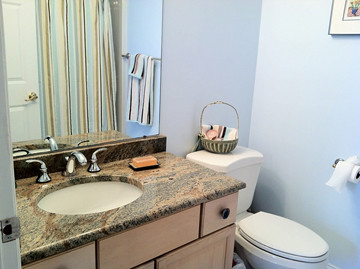This image captures an impeccably tidy and well-organized bathroom that exemplifies a seamless blend of modern and classic design elements. The centerpiece is a chic light-colored wood cabinet adorned with sleek, bronze-toned handles and contemporary silver accents. The countertop is an exquisite blend of brown, caramel, and subtle black hues, creating a beautifully marbled effect. 

A matching set of silver, uniquely angled, smooth handles adorn both the cabinets and drawers, enhancing the bathroom's sophisticated aesthetic. Atop the countertop sits a stylish black tray, which holds an orange square bar of soap, adding a splash of color to the setting.

Reflecting in the pristine mirror is a set of striped shower curtains, featuring a harmonious mix of brown, blue, and white stripes. Echoing this pattern, a towel hangs neatly on a bar, also flaunting brown, blue, and white stripes. The walls are painted a soothing light blue, providing a calm, airy feel to the room. 

Adjacent to the wall is a standard white toilet with an elongated seat. On its tank sits a small basket in a light brown or gray shade, containing a washcloth that matches the striped towel. Within this basket, a small, round object is tucked away.

In the upper right corner of the image is a professionally matted photograph of flowers, framed in a slim metallic frame, adding a touch of elegance to the restroom. Additionally, there is a roll of toilet paper mounted on a sleek silver holder, completing the bathroom’s tidy and cohesive look.